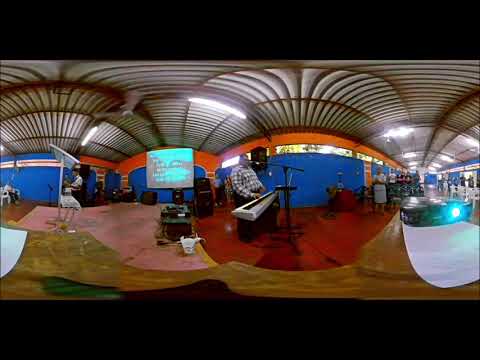In the image, a man in a checkered shirt is standing centrally, playing a white keyboard and possibly singing into a microphone. The venue, likely a church, features a scalloped white ceiling and a multicolored floor with shades of brown, pink, red, green, and white. Behind the pianist, a large screen, possibly 80 to 90 inches wide, suggests advertisements or presentations. The room's walls are primarily blue with orange accents, and there is ample space for movement. To the man's right, a small group of people listens attentively, while another person stands at a keyboard on the left. The atmosphere is illuminated by blue lighting, hinting at an event where people might be dancing or clapping, enhancing the lively and communal ambiance of the space.